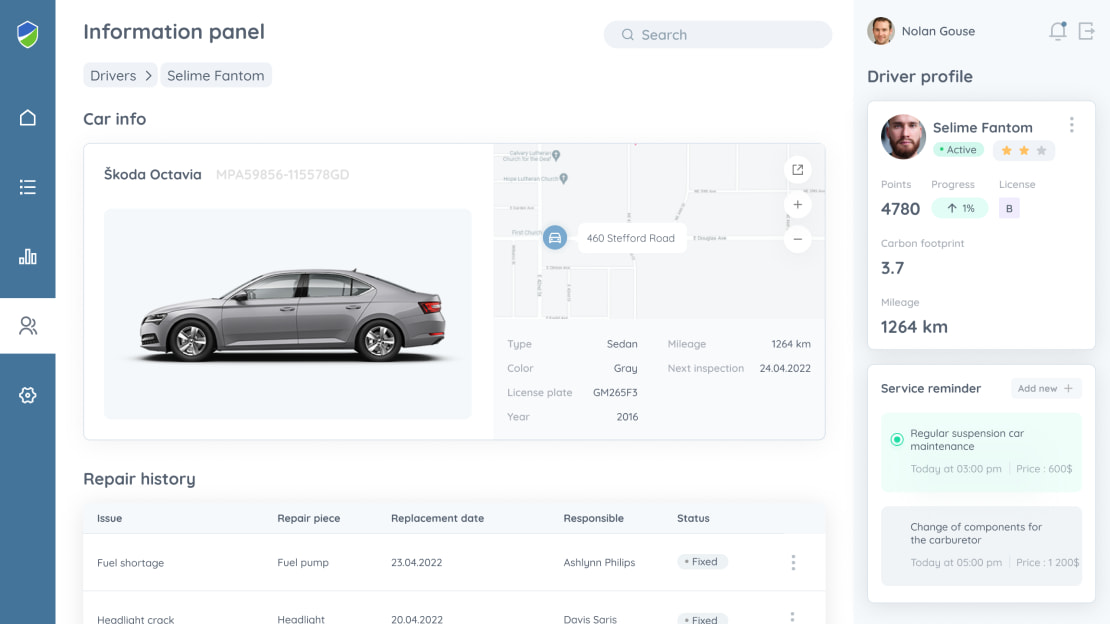**Detailed Caption:**

The image features a detailed screen displaying information about a gray, four-door Skoda Octavia sedan. This brand-new looking sedan is equipped with various features and navigational symbols on the left-hand side, including a coat of arms, a house, three lines, a cityscape, and stick-figure-like icons representing a person. Additional symbols include one resembling a snowflake or lotus and another depicting a box with a circle and dot in the center.

The top section of the screen includes a search bar with a magnifying glass icon and the word "Search." The main information panel, which occupies about three-quarters of the screen's width, provides comprehensive details about the car. 

On the far right of the screen, there's a profile picture labeled "Driver Profile: Seleney Phantom" alongside a photo and contact details for Nolan Gauss. The screen also displays icons that resemble a bell with a dot and a document with an arrow.

Key details about the Skoda Octavia include:
- **Vehicle Type:** Sedan
- **Mileage:** 1,264 kilometers
- **Color:** Gray
- **Next Inspection Date:** 24-04-2022
- **License Plate:** GM (partial details provided)
- **Year:** 2016

Despite its 2016 manufacture date, the car has surprisingly low mileage, hinting at either minimal usage or a potential data error. The car's detail panel also includes a history of repairs:
1. **Repair:** Fuel shortage
   - **Part Repaired:** Fuel Pump
   - **Repair Technician:** Ashlyn Phillips
2. **Repair:** Headlight crack
   - **Part Replaced:** Headlight
   - **Repair Technician:** Davis Saris
   - **Status:** Fixed (2022)

This detailed information screen offers a comprehensive overview of the vehicle's features, history, and status, emphasizing both its current condition and maintenance record.